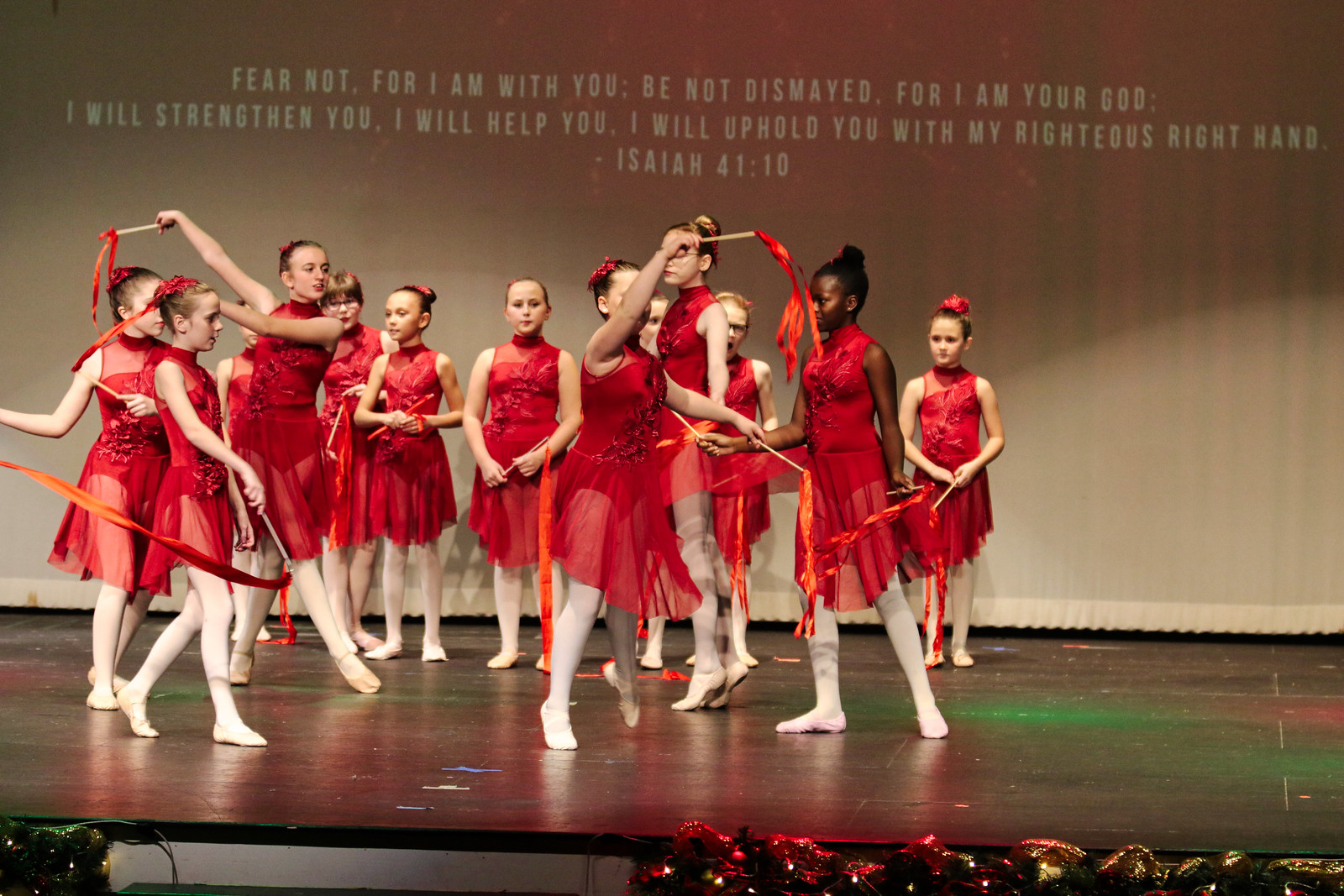The image depicts a performance by twelve young girls, approximately 12 years old, on a brightly lit stage. Eleven of the girls are Caucasian, and one, positioned second from the right, is Black. They are dressed uniformly in knee-length red dresses, white stockings, and white ballet shoes, with their hair styled in buns adorned with red bows. The girls are in various stages of dynamic movement, each waving a baton with streamers attached. Above them, a projector screen displays a biblical quote: "Fear not, for I am with you. Be not dismayed, for I am your God. I will strengthen you. I will help you. I will uphold you with my righteous right hand." - Isaiah 41:10.